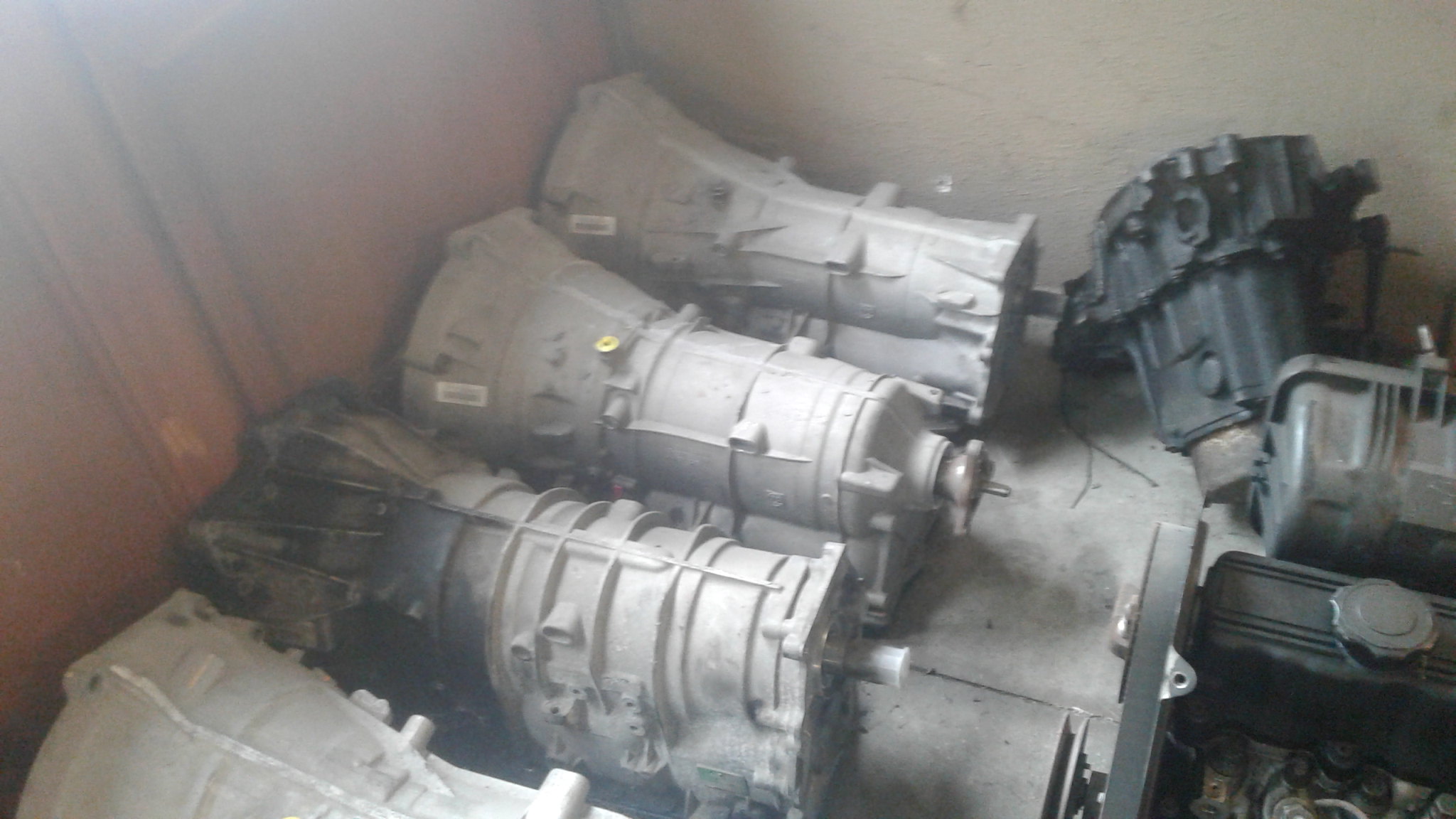The photograph captures an interior space, possibly a garage or machinery workshop, defined by a gray concrete floor and featuring a combination of a brown wooden wall on the left and a white or gray wall on the right. Aligned against these walls are at least four metallic or plastic devices, potentially some type of machinery or engines, all similarly coated in a fine layer of dust, giving them a uniformly grayish appearance. A closer look reveals barcodes on two of these devices that are positioned near the corner where the walls meet. These objects, mostly cylindrical with slightly flared ends, might resemble stage lights, microscopes, or flashlight handles. One of these devices notably has black areas peeking through the dust layer. The right edge of the image captures a glimpse of a heavy-duty storage case, hinting at the functional nature of the space. Shadows and lighting variations obscure some details, adding to the visual complexity of the scene.